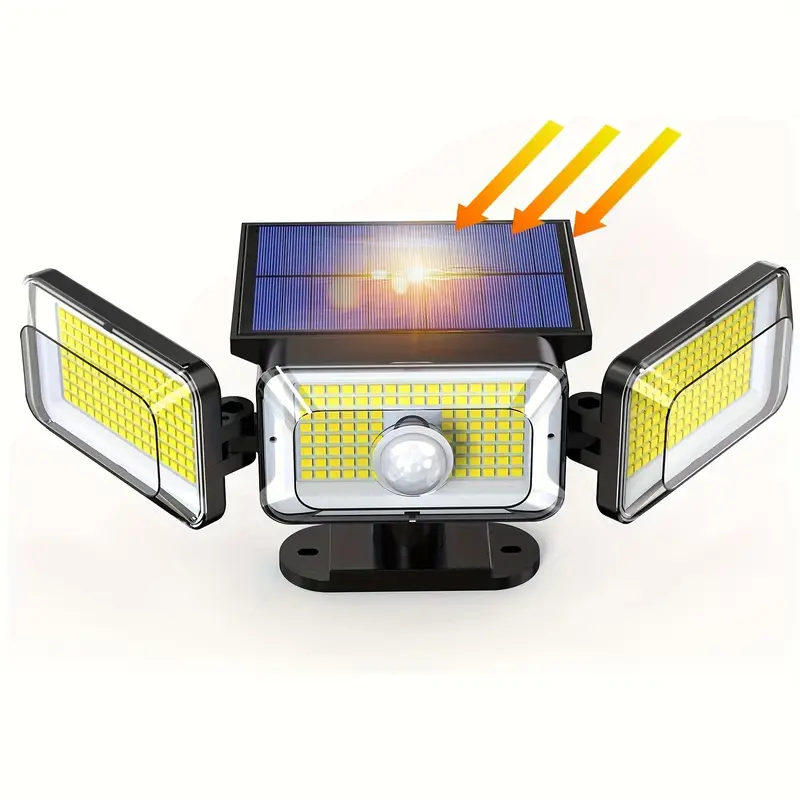This detailed rendering showcases a solar-powered work light featuring three adjustable LED lights. The central light is fixed, while the two side lights are attached to pivoting arms, allowing for customizable lighting direction — one aimed forward, one to the left, and one to the right. Mounted at the top is a large solar panel responsible for harnessing sunlight to power the LEDs, as indicated by three yellow-orange arrows representing sun rays converging on the panel. The lights are supported by a bracket, which appears suitable for mounting, and the background is entirely white, emphasizing the device's design. Additionally, the central light contains what seems to be a sensor, suggesting it might activate only in low light conditions.